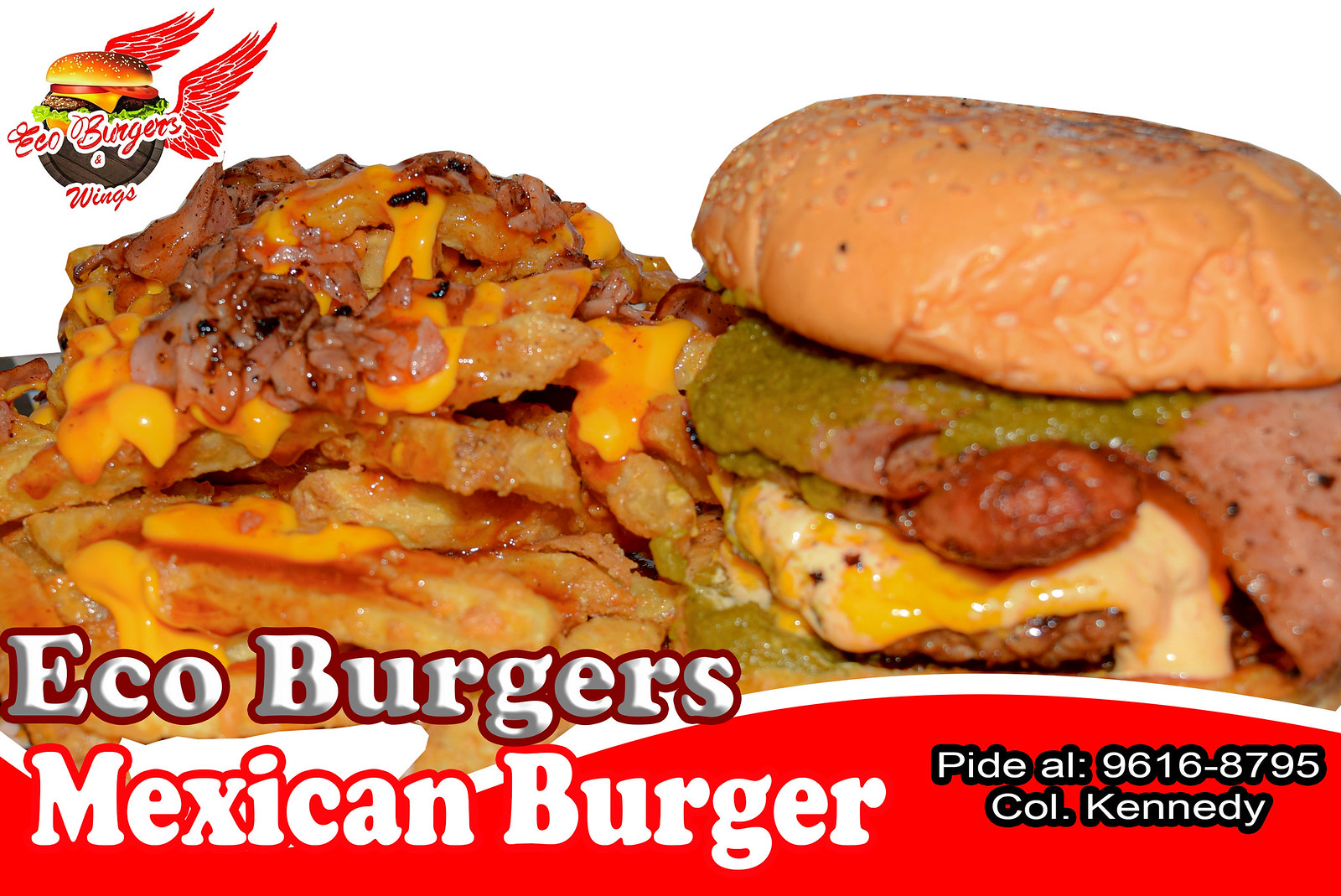This is a detailed advertisement image for Eagle Burgers and Wings featuring a prominent red background. In the top left corner, there is an animated icon of a burger with red angel wings and the text "Eagle Burgers and Wings" across it. The focal point of the ad is a detailed picture of a meal: crispy french fries generously topped with melted cheese, a rich meat sauce, and sprinkled with onions. Beside the fries is a hefty burger featuring a golden bun, layers of bacon, beef patty, melted cheese, and a distinctive green sauce, possibly guacamole or a special condiment. Notably, the burger also appears to contain an egg. In the lower left corner, the text reads "Eagle Burgers," followed by "Mexican Burgers" on the next line. The lower right corner includes a contact detail "Pied Al. 9616-8795" and mentions "COL. Kennedy." The advertisement suggests a theme of indulgent, saucy, and flavorful Mexican-inspired burgers that promise a hearty meal experience.